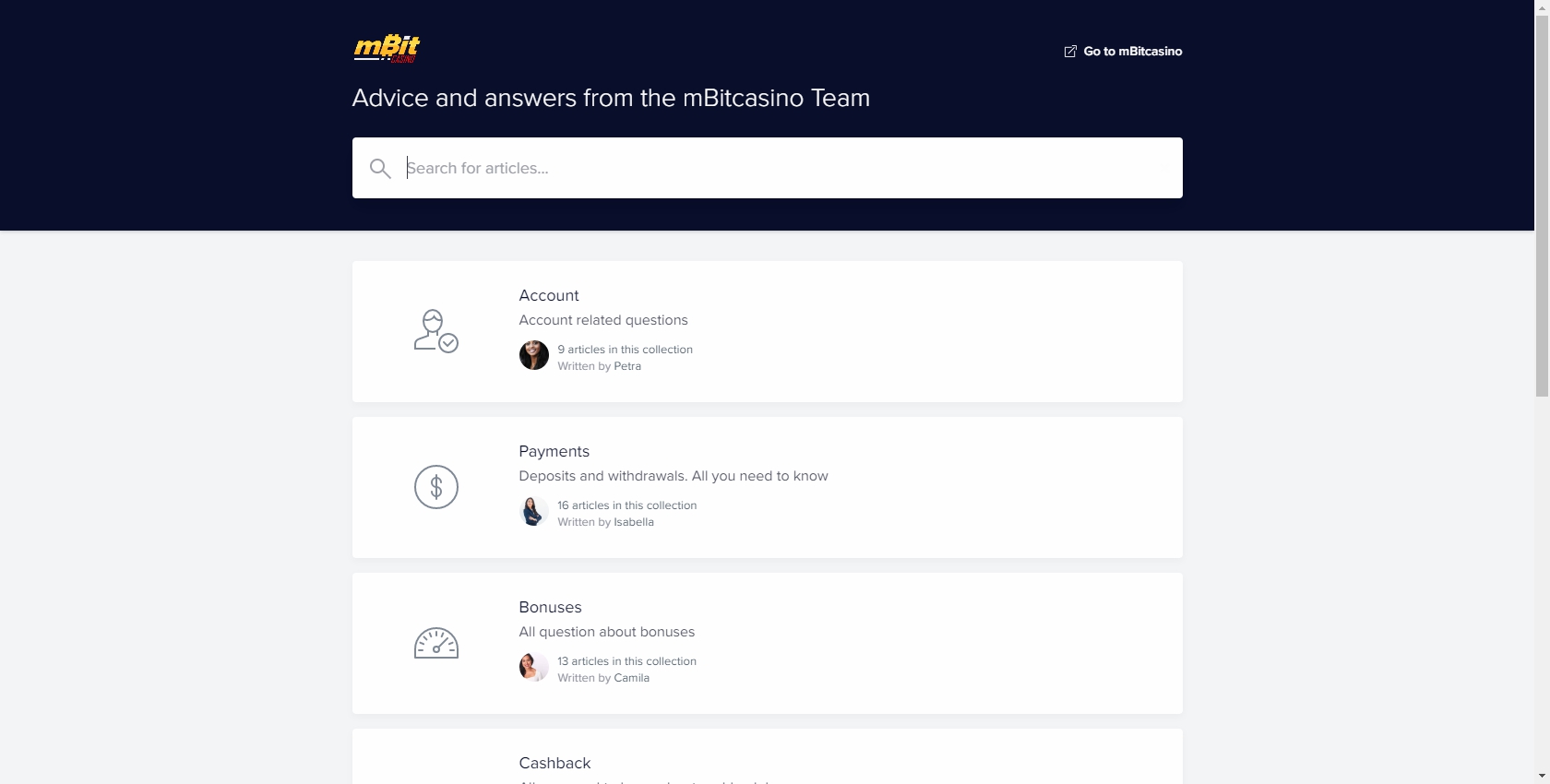This is a left-to-right horizontal website image, typical of a computer or smart device interface. The layout features a dark gray or dull black rectangular banner stretching across the top of the screen. Within this banner on the middle left, there is yellow text displaying "MBIT." Directly beneath this, a tagline reads, "Advice and Answers from the MBIT Casino Team."

Towards the right center of the screen, there is a prominent white box with a checkmark icon and text that reads, "Go to MBIT Casino." Below the tagline, there is a white search bar with a magnifying glass icon, inviting users to "Search for Articles."

The main content of the page is organized within a light gray box, populated with several white rectangular sections, each featuring text and various icons. The first section includes a person icon with a checkmark and is labeled "Account: Account-Related Questions," containing nine articles authored by a patron. The second section displays a dollar sign icon and is titled "Payments: Deposits, and Withdrawals, All You Need to Know," with sixteen articles written by Isabella.

The third section is dedicated to "Bonuses: All Questions About Bonuses," featuring thirteen articles written by Camilla, accompanied by a relevant icon. Below this, there is another section that begins with "Cashback," but the content of this section is not fully visible.